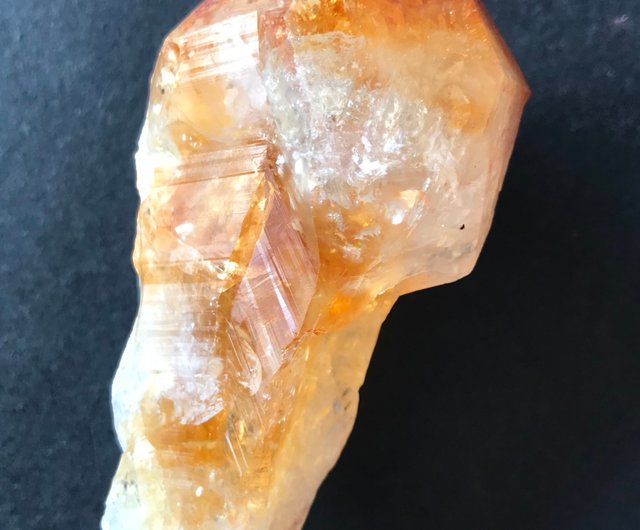The image depicts a close-up of a shiny, gem-like rock set against a black background that lends a dramatic contrast to the subject. The rock itself features an intriguing mixture of colors—primarily vibrant oranges and pristine whites, with occasional pink and brown specks, and subtle black inclusions. Its intricate structure reveals clear sections that allow light to penetrate, enhancing its glossy appearance. The rock's shape is somewhat spherical at the top, tapering toward the bottom, resembling a pole-mounted ornament. The surface of the rock is uneven, adorned with streaks of white that traverse both vertically and horizontally, adding to its unique and captivating texture.